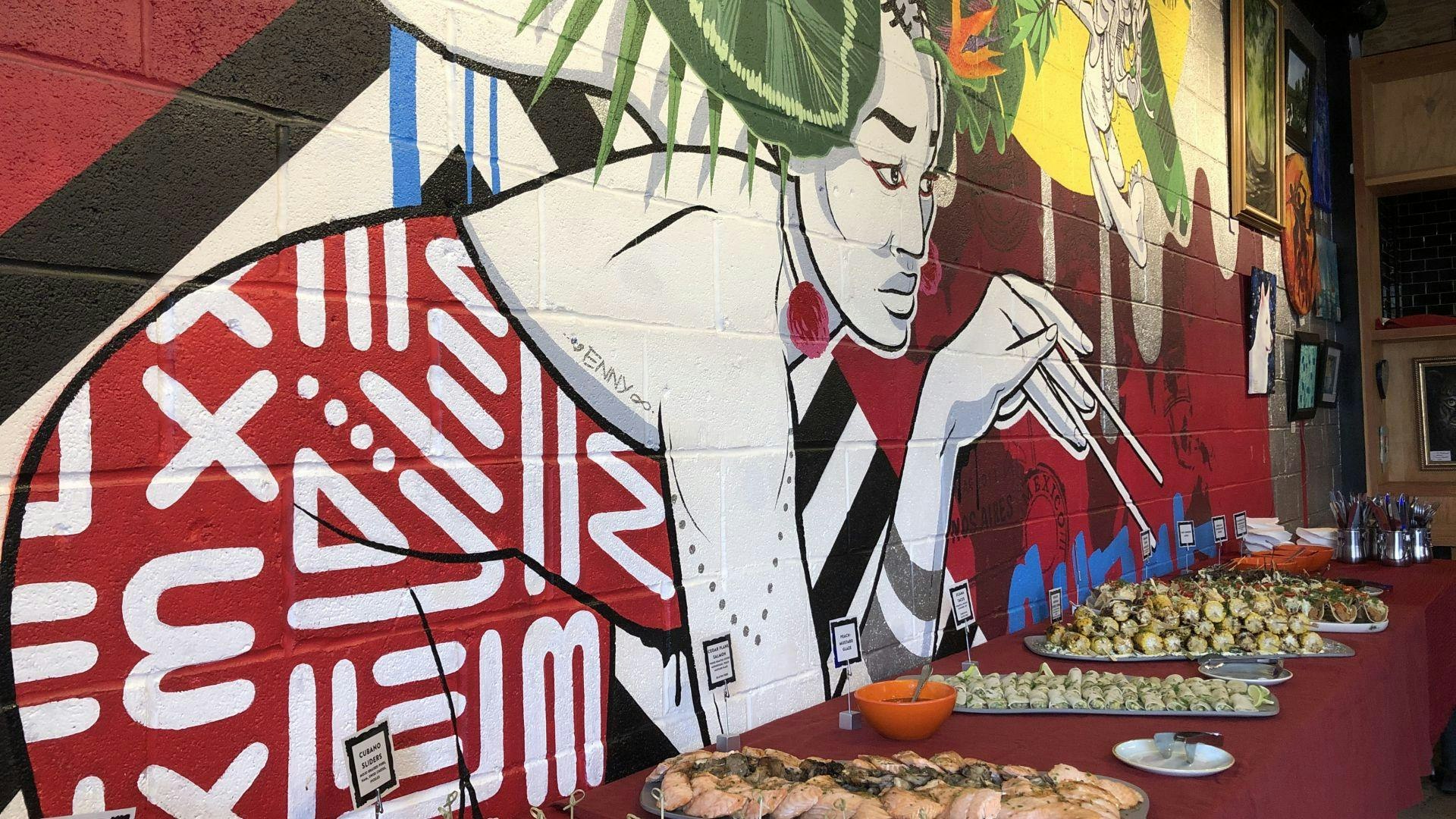The photograph captures a vividly painted indoor cinderblock wall featuring an intricate mural. Dominating the mural is an Oriental woman, dressed in a red and white attire, bent over with chopsticks in her left hand, seemingly reaching for the food on a table positioned in front of the wall. Her attire, resembling a sari, bears white letters and lines, and foliage encircles her head. Behind her, the wall boasts a striking red background, a black triangle with a white triangle underneath, and intricate details of green leaves. Adjacent to her, a large bird with green feathers and a gray body extends across the wall.

In front of this colorful mural, a long table is adorned with a maroon tablecloth, laden with oblong trays of various foods and an orange bowl with spoons sticking out of it. At the far end of the table, silver cups filled with silverware and a stack of white napkins can be seen, completing the detailed setting. The artist's skillful placement of the woman makes it appear as though she is about to pick up food from the trays, blending art with reality in a striking, creative scene.